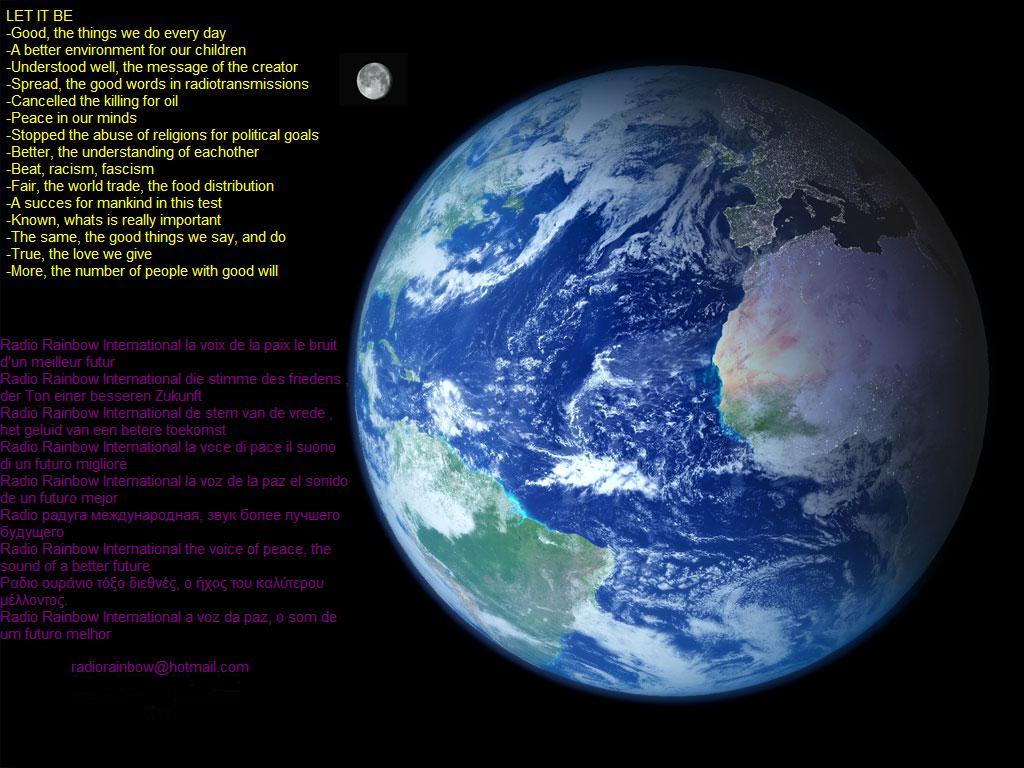The image features a predominantly black poster or slide with a detailed composition. On the left side, a vertical column showcases yellow text against the dark background. At the top of this yellow text column, the phrase "let it be" is displayed, followed by a hyphen with several lines of text beneath it. The text reads, "let it be good the things we do every day, a better environment for our children, understood well the message of the creator, spread the good words in radio transmissions, cancel the killing for oil, peace in our minds, stop the abuse of religions for political goals, better the understanding of each other, beat racism, fascism, fair the world trade, the food distribution, a success for mankind in this test, known what is really important, the same the good things we say and do, true the love we give, more the number of people will with goodwill." Below this yellow text, a paragraph in purple font further elaborates on these themes.

To the right side of the poster, a vivid picture of planet Earth is prominently displayed, showcasing its blue, green, and yellow hues. In comparison to the Earth, a small white planet, possibly representing the moon, appears between the text column and Earth, adding to the cosmic theme of the poster. The carefully curated text and imagery collectively emphasize themes of environmentalism, peace, understanding, and global unity.